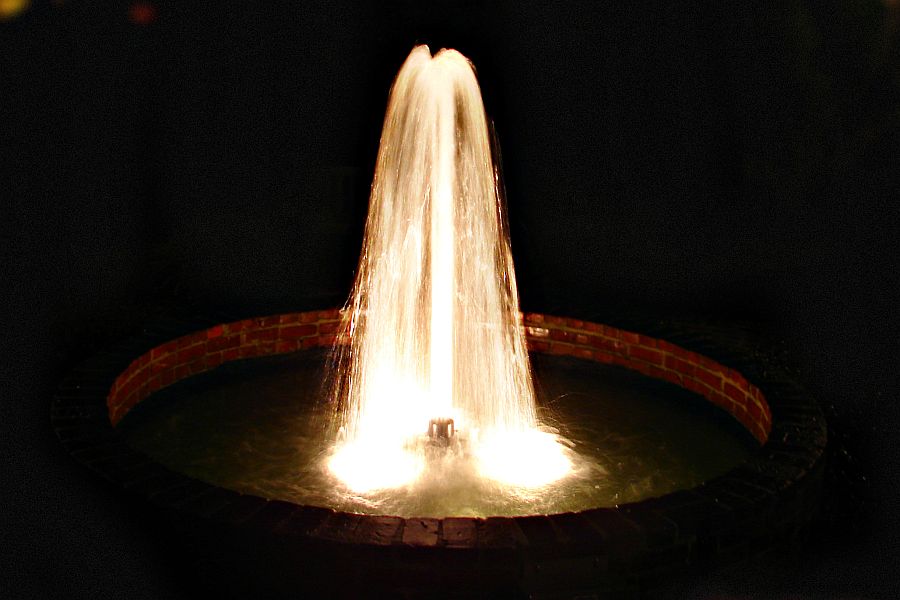This nighttime photograph captures a mesmerizing scene of a lighted water fountain. The backdrop is pitch black, highlighting the luminescent feature at the center. Set within a large circular basin constructed from vibrant red bricks, a serene pool of water serves as the fountain's focal point. From the center of this pool, a cylindrical pump propels water upwards in a dynamic spray, which cascades gracefully back into the basin. The fountain is bathed in a radiant yellow light, causing the water to glow brilliantly and creating a striking contrast against the dark surroundings. The overall effect is both enchanting and tranquil, showcasing the beauty of illuminated water features in the night.